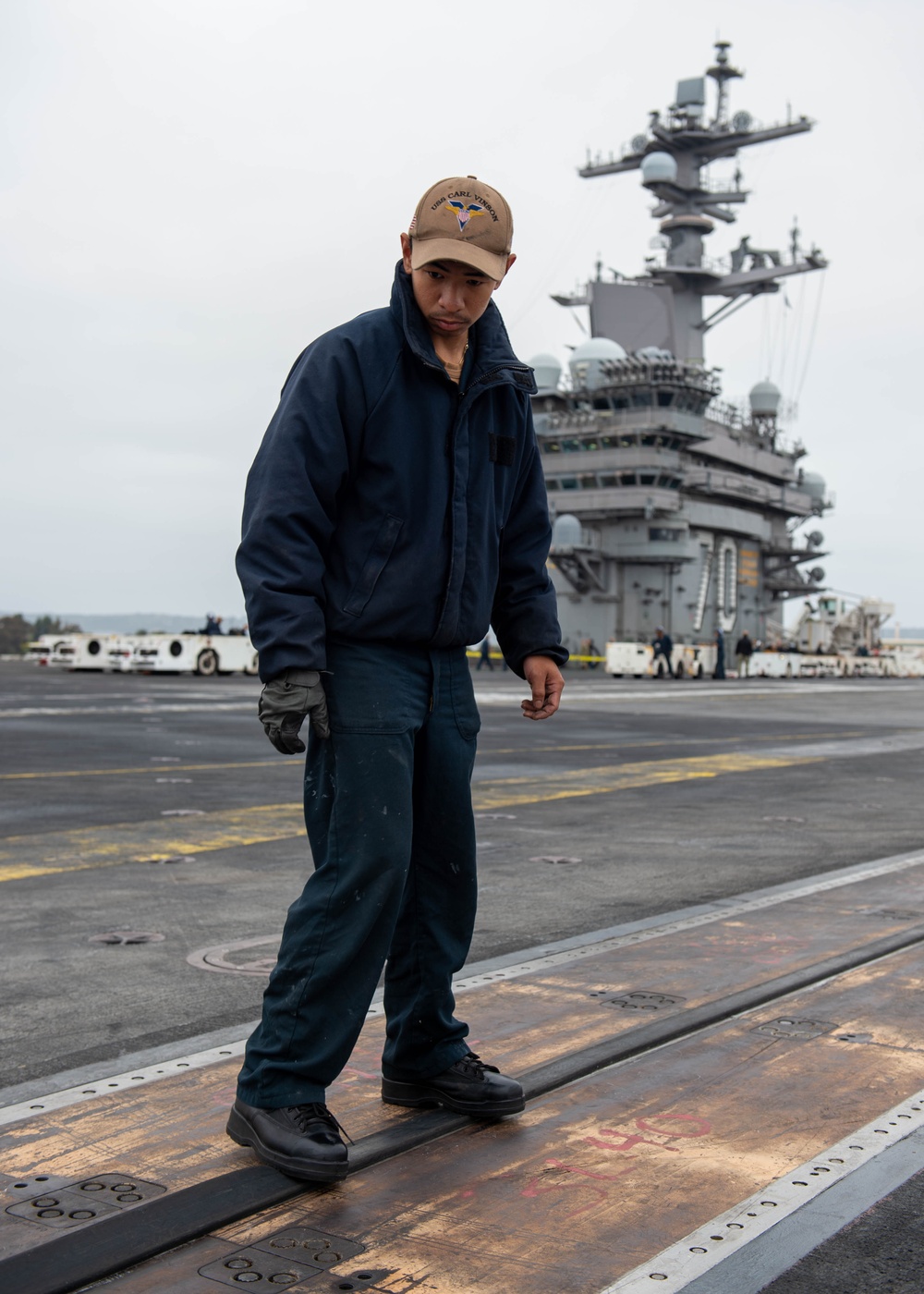A young dark-complected Asian man stands prominently on the deck of an aircraft carrier, positioned at the center of the photograph. He is attentively looking downwards, immersed in his task. He sports a dark blue work jumpsuit and heavy black boots, complemented by a grey glove on his right hand, while his left hand remains bare. Crowning his look is a tan trucker cap with an unreadable insignia, likely related to the USS Carl Vinson, the ship's name. The deck beneath him, partially covered by a reflective metal strip, extends from the bottom right to the bottom left of the image. This metal strip lies on the black tarmac marked with yellow lines. In the background, the ship's air traffic control tower, radar masts, and aerials punctuate the scene, evoking the intricate and modern workings of a naval vessel. To the left of the control tower are several small transport vehicles, suggesting the tools used to move aircraft around the carrier's deck. The overall setting bears an industrial and functional ambiance, underscoring the diligent atmosphere of the aircraft carrier.